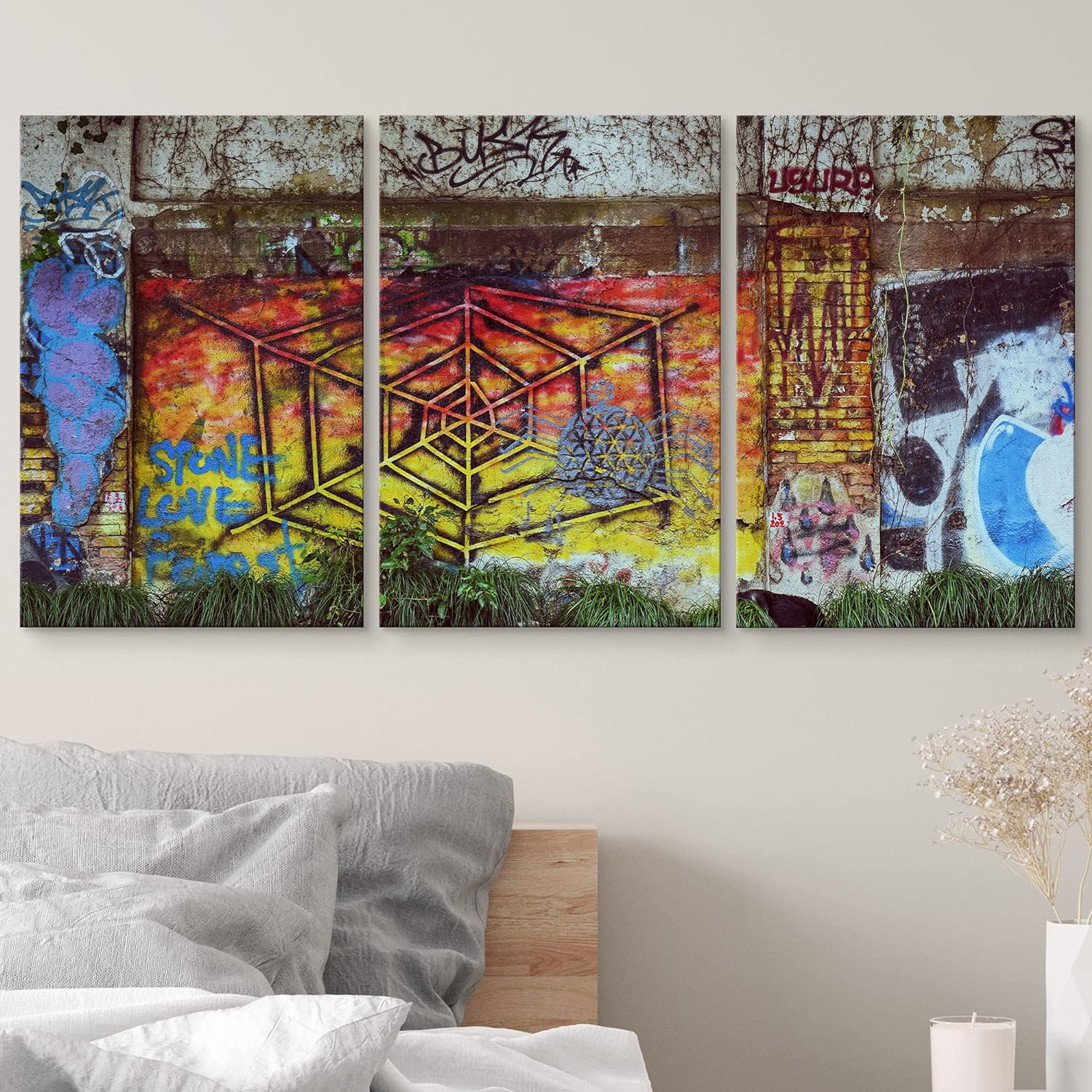This detailed photograph captures the interior of a bedroom, prominently showcasing a unique, artistic wall. The focal point is a triptych mural, depicting an abstract spider web design in bold yellows and reds, spanning from the left panel through the middle and concluding on the right panel. The mural, set against the textured backdrop of a white concrete wall, is vividly adorned with various graffiti elements, including blue patterns and textual components. Adjacent to this striking artwork, on the bottom left, is part of a bed frame with light brownish-cream bedding complemented by white pillows. The right bottom corner features a serene arrangement of a white candle and a dried flower vase, adding an elegant touch to the vibrant and eclectic decor of the room.